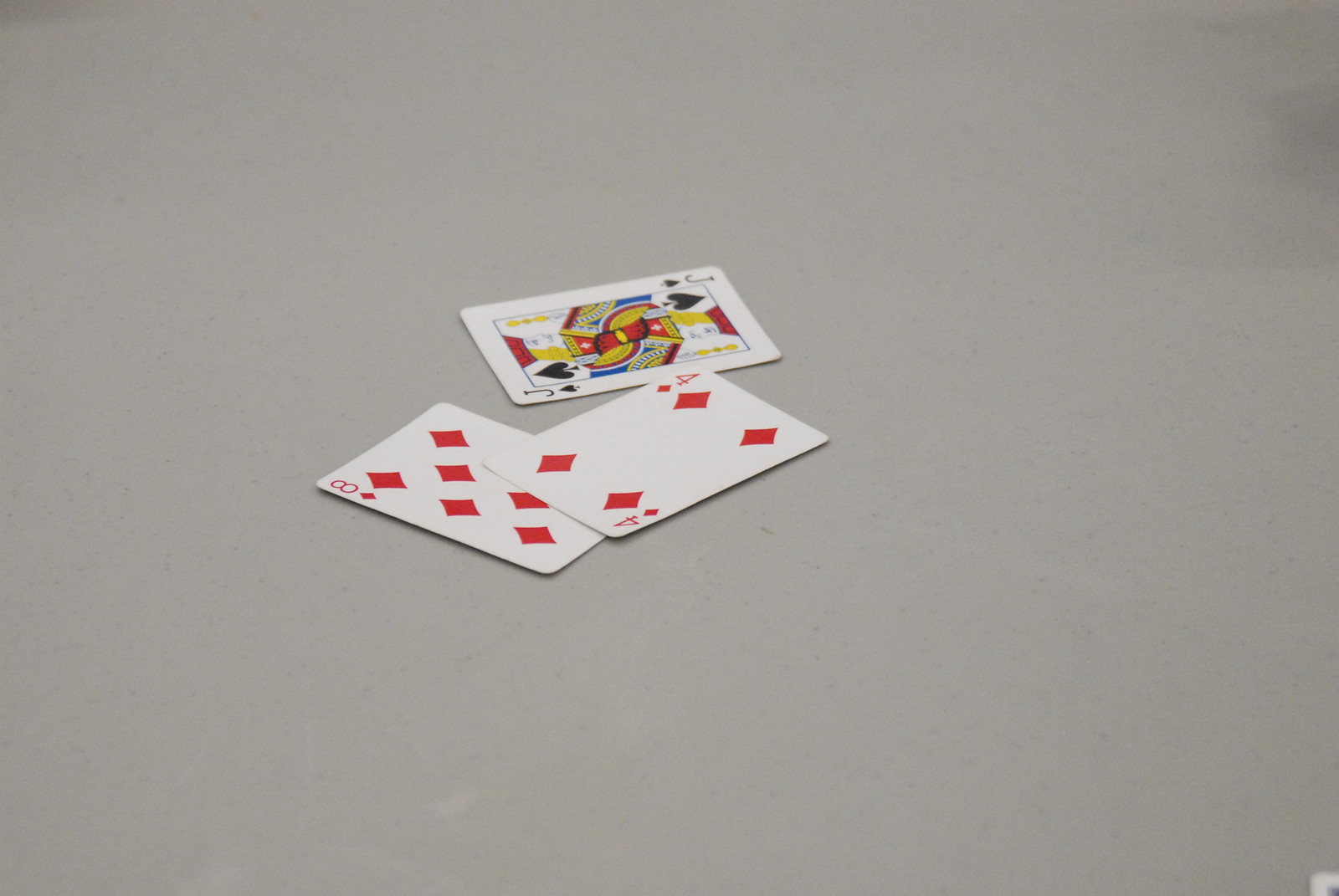The image features three playing cards laid face up on a grey background. The first card, positioned on the left, is the Eight of Diamonds. It is adorned with eight red diamonds, although only six are visible as two are partially obscured by another card. The number "8" is displayed in red at the top left and bottom right corners, each accompanied by a small red diamond symbol.

The second card, the Four of Diamonds, sits partially over the bottom of the Eight of Diamonds. It prominently displays the number "4" in red at the top left and bottom right corners, with a small red diamond under each. Four larger red diamonds are positioned in a 2-2 pattern on the card's face—two at the top and two at the bottom.

The third card, a Jack of Spades, is placed slightly in front and beneath the Four of Diamonds. This card features a black "J" in the top left and bottom right corners, along with a black spade symbol. The spade is depicted as an upside-down heart with a stem. The Jack's design includes a mirrored image of a crowned figure with golden hair, wearing a robe in shades of red, blue, and yellow. The figure holds a staff with a golden tip.

A faint shadow is visible in the top right corner of the image, adding depth. Additionally, the bottom right corner reveals the edge of another card, hinting at more cards beyond the frame.